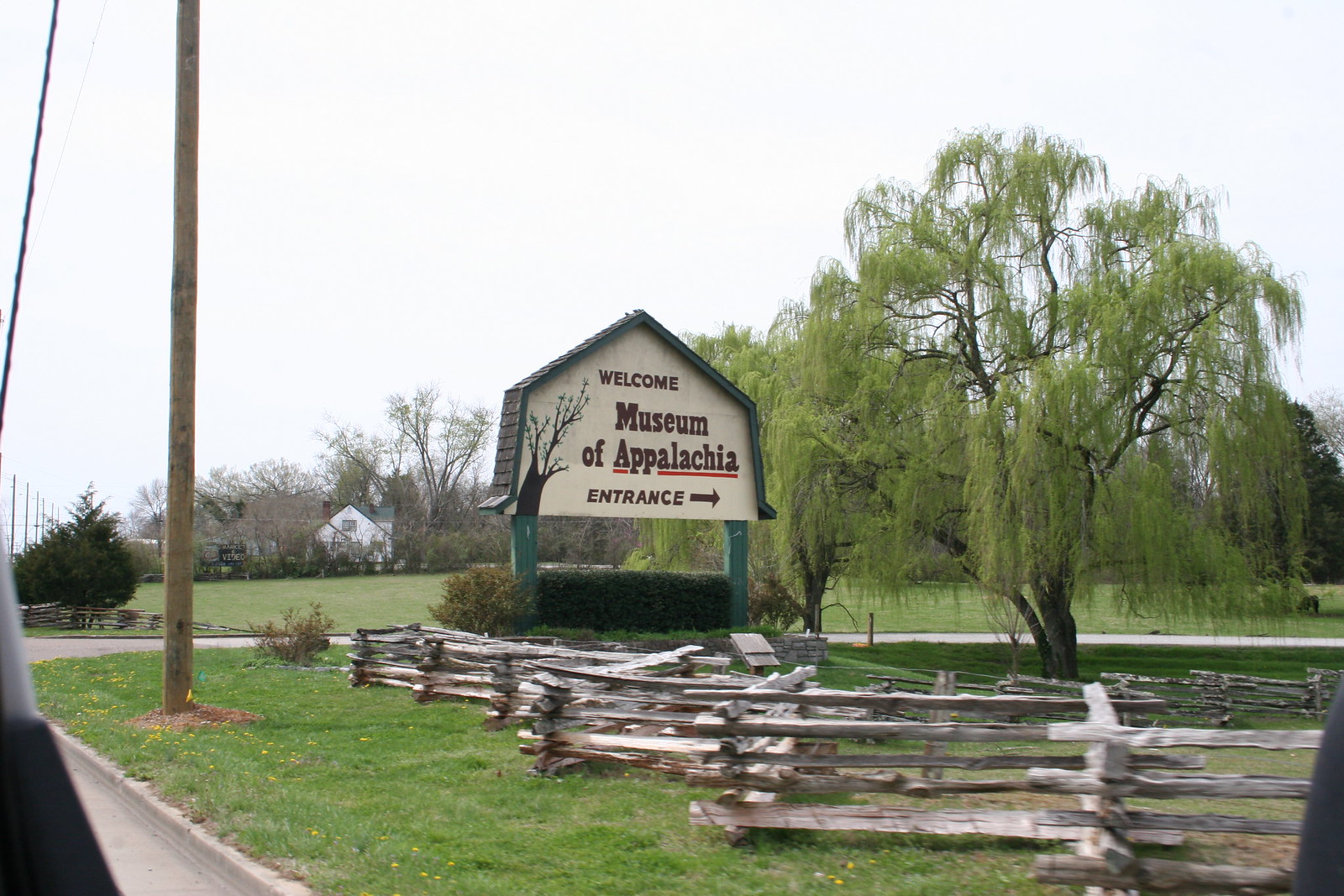The image showcases a wide, rectangular scene of an entrance to the Museum of Appalachia. Dominating the foreground is a large, well-manicured grassy area enclosed by a zigzagging wooden fence. Central to the image is an off-white sign, fashioned in the shape of a house with green wooden posts and a brown roof-like border. The sign features a drawing of a tree with green leaves on the left and reads in brown font, "Welcome Museum of Appalachia Entrance," with "Appalachia" underlined in red paint and an arrow pointing to the right. A massive green tree occupies the right corner of the image, complementing the greenery of the grassy area. Further details include a background filled with additional trees, a road leading into the distance, a weathered white house, and a telephone pole. The scene is bathed in daylight, and no people can be seen in this tranquil setting.